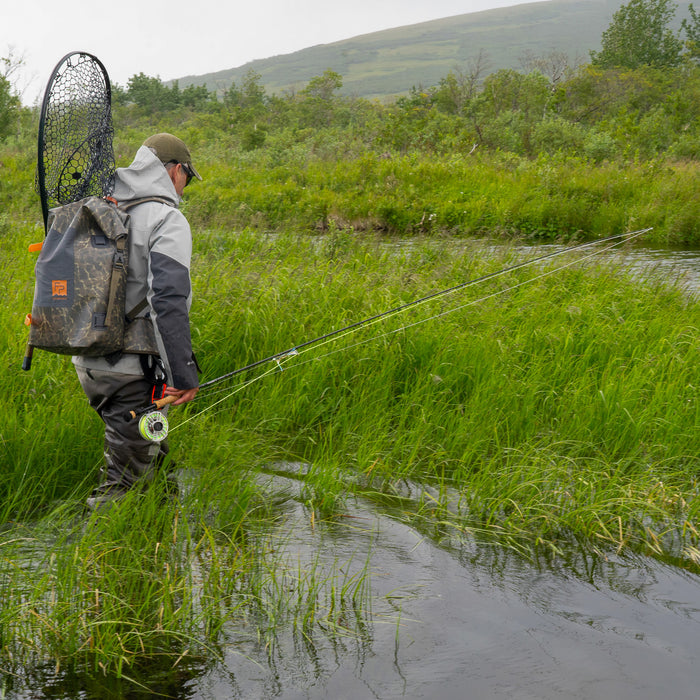This image captures a serene nature scene featuring a fly fisherman standing in the left side of the frame, facing right, with his back turned to the camera. The fisherman, who cannot be seen from the front, is dressed in a light grey hooded parka with dark grey sleeves and a nice, camouflage grey backpack accented with orange trim. He’s wearing greyish-green pants and knee-high boots, partially submerged in swampy water, surrounded by tall, waist-high grasses. A large black fishnet is strapped to his backpack with gold-orange straps, hanging over it. In his right hand, he delicately holds a long, approximately 12-foot fly fishing rod, made of simple black graphite with a bright green leader cable. The day appears to be overcast, possibly taken in the afternoon, lending a diffuse light over the lush green scene filled with grass and trees. Although the image is vibrant, there is no text or photographer's signature visible. The fisherman appears poised, as if aiming his lure towards another body of water beyond the immediate frame.